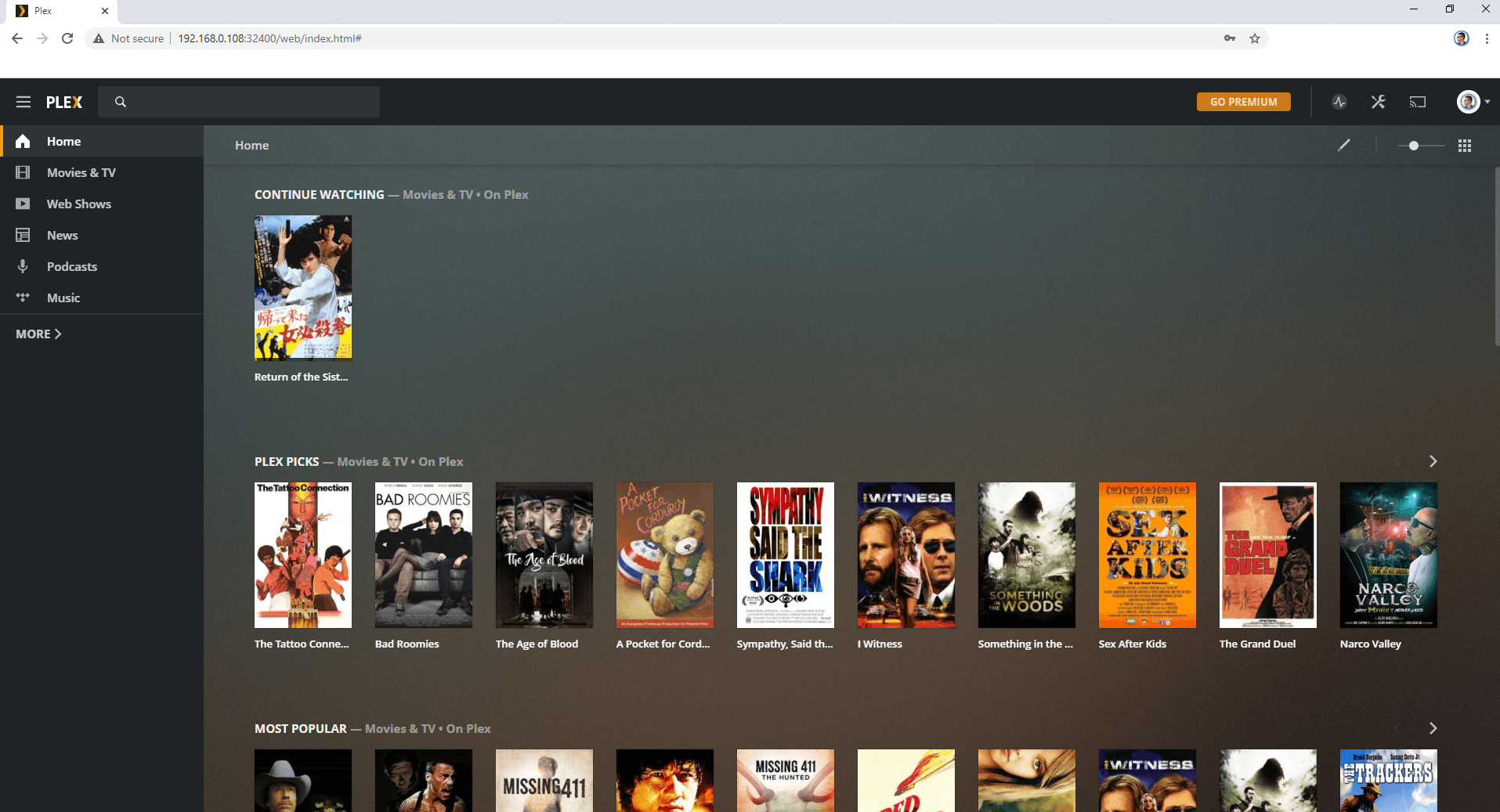This image is a screenshot of the Plex website. In the upper left corner, there's the Plex folder tab icon followed by the word "Plex". To the right is a close button (X). Below this, a gray left-pointing arrow, a light gray right-pointing arrow, and a refresh icon are visible. 

Directly below, an address bar shows that the connection is “Not Secure,” with the URL displayed next to a key icon and a star icon on the right.

A black banner beneath the address bar features a hamburger menu icon followed by "Plex" and a magnifying glass search icon to the left. On the right side of the banner, there's a "Go Premium" button and several other icons.

Highlighted on the left sidebar is the home icon, with options listed below for "Movies & TV," "Web Shows," "News," "Podcasts," and "Music." Further down, an option for "More" with a right-pointing arrow is available.

In the main content area, to the right of the sidebar, it says "Home." Below this, under "Continue Watching," there's a section for "Movies & TV," showing a thumbnail of a movie with an unclear title. Further down, there’s a "Plex Picks" section with a row of movie thumbnails. Lastly, a partially visible section for "Most Popular" is also seen, featuring additional media images.